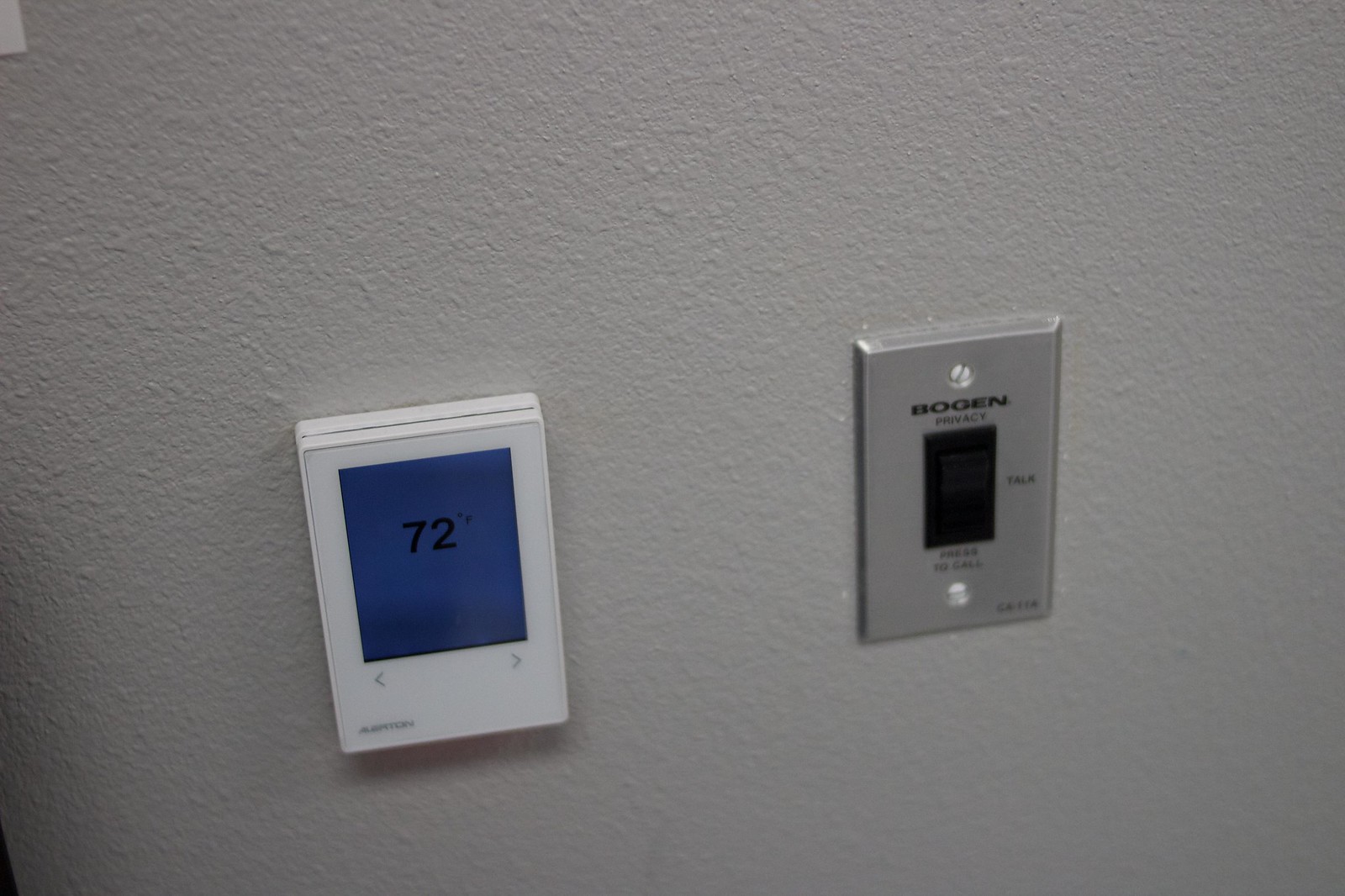In this indoor photograph, a white textured wall prominently features a sleek thermostat and an intercom switch. The thermostat, which is white with a blue digital display, clearly shows the temperature set at 72 degrees Fahrenheit in black numerals. Beneath the display are two navigation arrows, one pointing left and the other pointing right, possibly for adjusting the temperature settings. 

To the right of the thermostat, a stainless steel switch plate branded with the name "Bogan" houses an intercom switch. This plate incorporates a black switch centered in its middle, labeled "TALK" in black lettering. The top and bottom of the switch have additional text that is not legible in the photograph. The switch plate is affixed to the wall with white painted, slotted screws, contributing to the clean and orderly appearance of the setup.